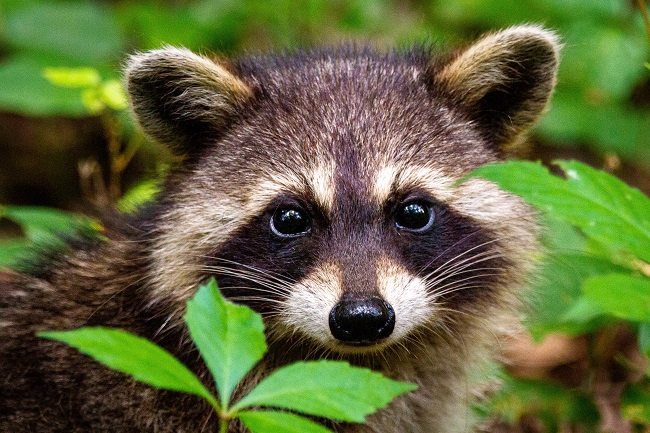In this close-up portrait, a young raccoon gazes directly at the camera, exuding a sense of innocence. The raccoon's face features a mix of black and white fur, with strikingly deep black eyes that sparkle with curiosity. Its snout is predominantly white, while the small nose contrasts sharply with its dark, wet shine and noticeable whiskers. The animal’s ears show a distinctive coloration—white on the outside and black on the inside. The image captures just the head and a bit of the neck and back, as the raccoon is framed by green leafy plants on both sides. The background consists of blurred leaves and hints of yellow, suggesting a natural setting, likely photographed during a bright, high-contrast day. The overall high saturation and detailed focus on the raccoon's face make it look almost as if it's posing, adding to its cute and endearing appearance.